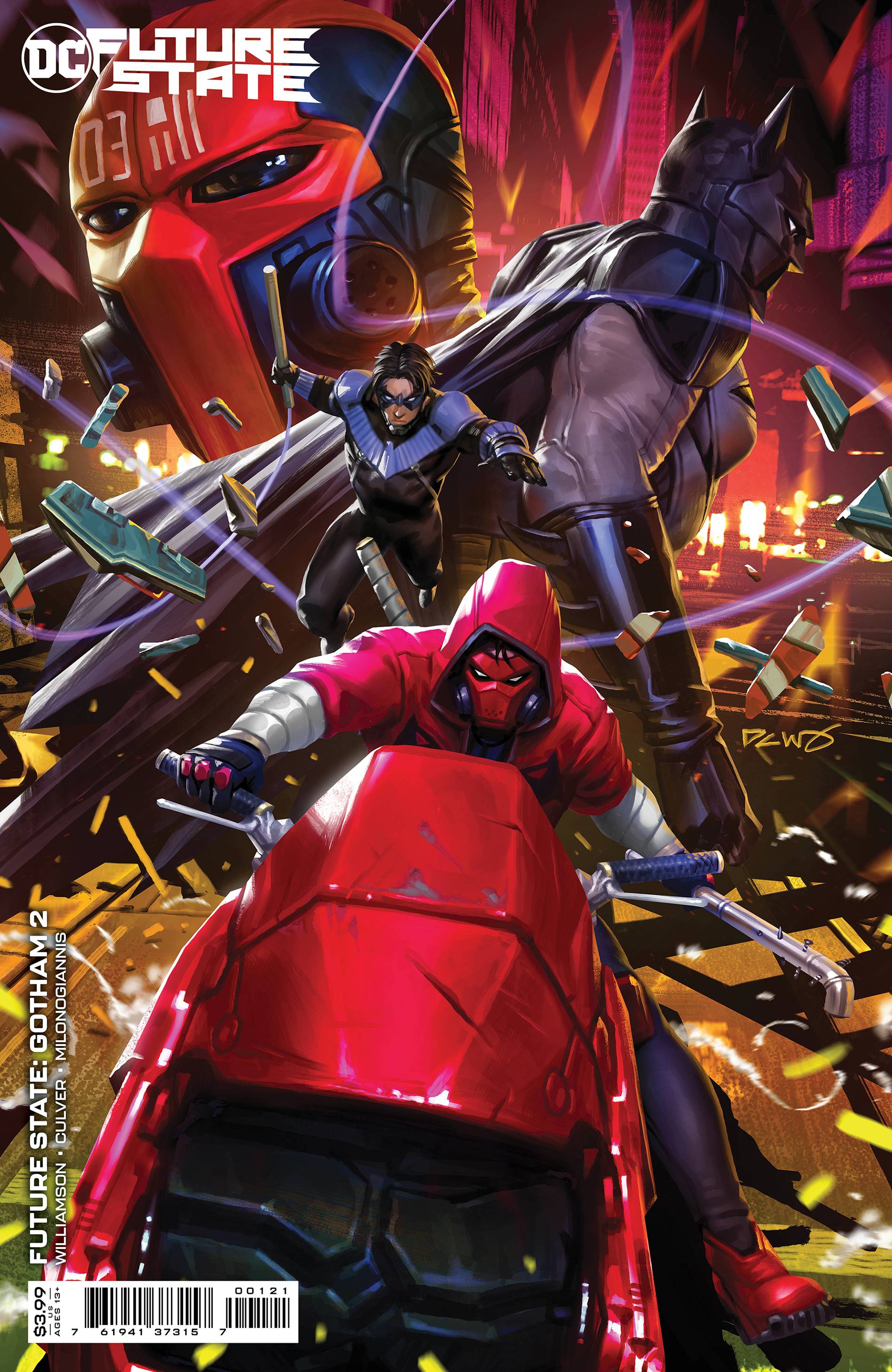This is the cover of a DC comic book titled "DC Future State: Gotham 2". The scene is packed with dynamic action and vibrant characters. At the top of the cover, "DC Future State" is written in prominent white font. The central figure is a superhero dressed entirely in red, including a red mask or helmet, red boots, and a red shirt. He is riding a red motorcycle, and he holds a club in his hand. Above him, there is a close-up of his red mask.

To the right, you can see Batman in a profile perspective, looking as if he's running or in motion. Below the central character on the motorcycle is Nightwing, easily recognizable in his black suit with blue details and a black mask. The left side of the cover features the title "Future State: Gotham 2", along with the creators' names—Williamson, Culver, and Milongians—and a UPC barcode beneath it. The cost of the comic is $3.99. The overall imagery conveys a sense of intense movement and excitement.